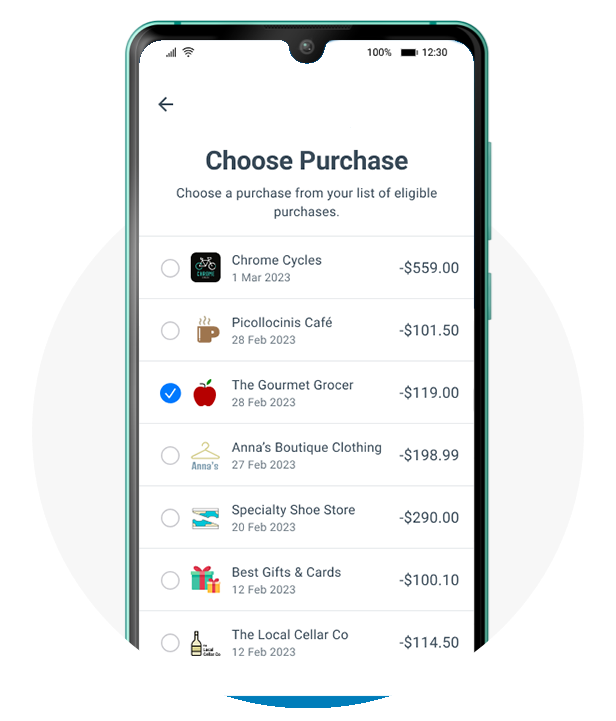Here's the cleaned-up and detailed caption:

---

The image resembles the home screen of a cell phone, framed by a green border with a darker black outline inside. At the top right corner, the battery icon displays 100% charge, and the time is shown as 12:30. 

Centralized text reads, "Choose Purchase" followed by the instruction, "Choose a purchase from your list of eligible purchases." Below this, a long gray line separates the instructions from the listed transactions.

The first transaction is in a black box labeled "Chrome Cycles" with the date "1 March 2023" underneath, showing a deduction of $559.00. 

Next, "Pilikulina Cafe" appears with a negative amount of $101.50, followed by a blue circle checkmark. 

Adjacent to an apple icon, "The Gourmet Grocer" shows a deduction of $119.00. Below this, "Anna's Boutique Clothing" displays a charge of $198.99.

Further down, "Specialty Shoe Store" lists a transaction dated "20th of February 2023" with a deduction of $290.00. Next is "Best Gifts and Cards" featuring a present icon with a red bow.

The final transaction at the bottom is from "The Local Cellar Company," accompanied by an image of a wine bottle and dated "12th, February 2023."

---